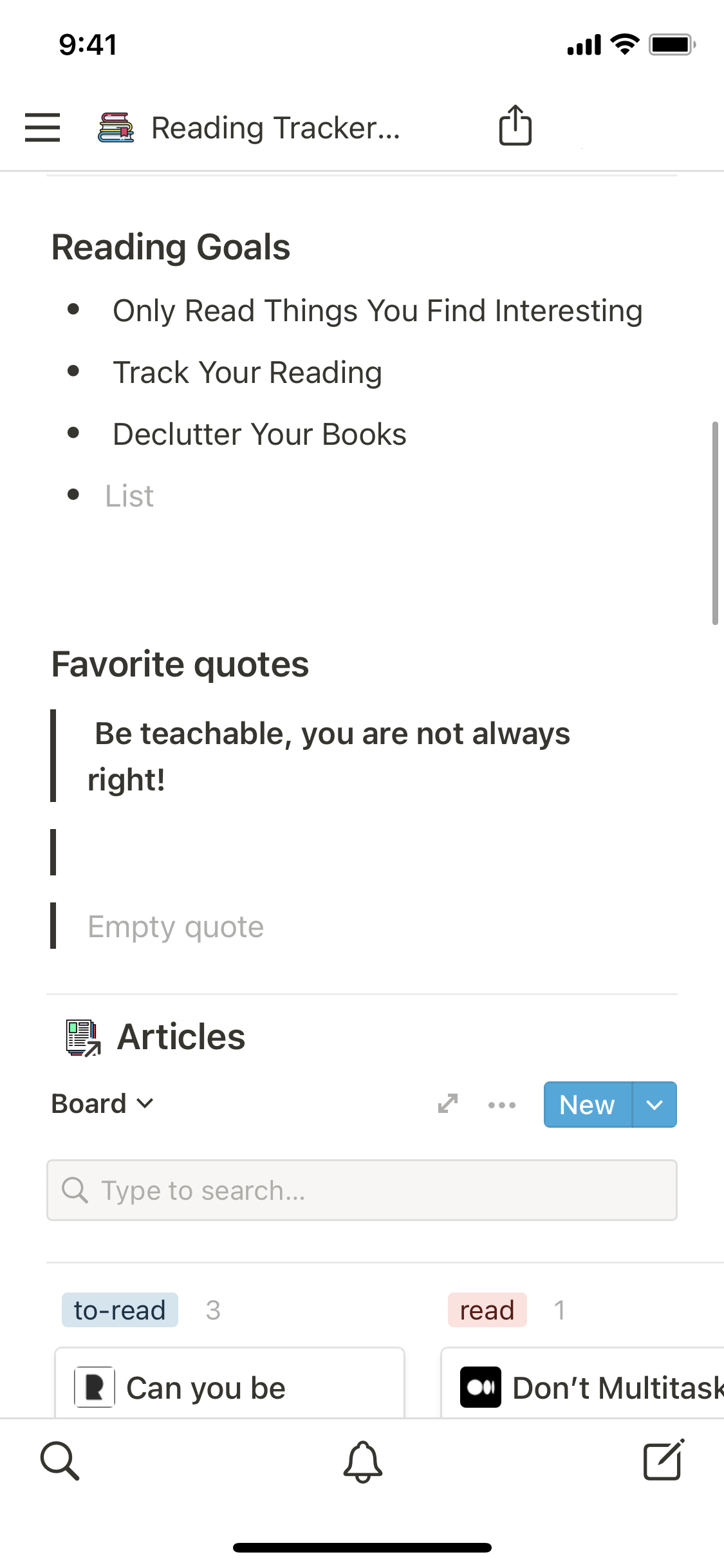A mobile screenshot captures a website interface featuring a white background with predominantly black text. At the top-left corner of the screen, the time reads "9:41." On the top-right, icons indicate full signal strength, Wi-Fi connectivity, and battery life. 

Below this, the page has a header with three horizontal lines (likely a menu icon) and a books icon, next to the title "Reading Tracker." Underneath the title, the section "Reading Goals" includes a bulleted list:
- Only read things you find interesting
- Track your reading
- Declutter your books

Following the goals section, in gray text, the word "List" appears. Further down, there's a section titled "Favorite Quotes," marked off by a horizontal line. Below this, a short quote reads: "Be teachable, you're not always right." Another line follows, with an empty quote section labeled "Empty Quote" in gray text.

Next, the "Articles" section appears with a dropdown menu labeled "Board," accompanied by a small gray arrow and three gray dots to the right. A blue rectangle features the word "New" in white with a downward arrow beside it. Below, there's a search bar with the placeholder text "Type your search."

On the main content area, the "To Read" section lists three items on the left-hand side, beginning with "You Can Be." On the right, in the "Read" section, the item "Don't Multitask" is noted.

At the bottom of the page are three icons: a magnifying glass on the left, a bell in the center, and a notepad symbol on the right. Below the bell icon lies a thin black line spanning about a quarter of the screen width.